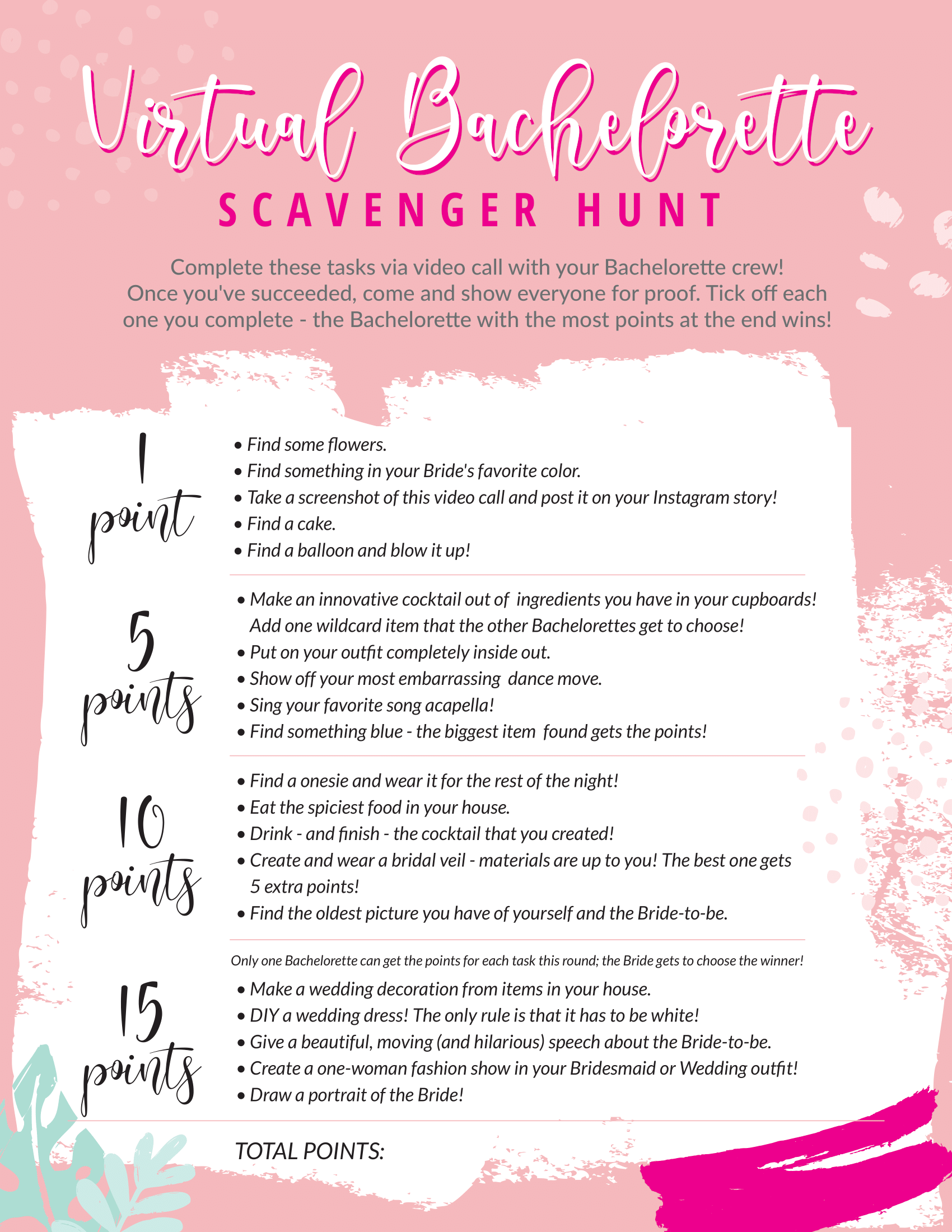The image displays a vibrant pink poster with a white center, designed as a detailed rule chart for a "Virtual Bachelorette Scavenger Hunt" game. At the top of the poster, the title "Virtual Bachelorette" stands out in a stylish white font with dark pink borders, followed by "Scavenger Hunt" in solid dark pink. Below the titles, green text instructs players to complete various tasks via video call with their bachelorette crew and to show proof of their achievements to earn points. The bachelorette with the most points at the end wins.

The white area in the center contains a structured list of tasks segmented by point values. Tasks include:

- **1 Point Tasks**: Find some flowers, find something in your bride's favorite color, take a screenshot of the video call and post it on Instagram, find a cake, find and blow up a balloon.
- **5 Point Tasks**: Make an innovative cocktail with ingredients from your cupboards, add a wild card item chosen by others, put on your outfit completely inside out, show off your most embarrassing dance move, sing your favorite song a cappella, find something blue, find a onesie and wear it for the rest of the night, eat the spiciest food in your house, finish your crafted cocktail.
- **10 Point Tasks**: Create and wear a bridal veil (materials up to you, best one gets 5 extra points), find the oldest picture with the bride-to-be.
- **15 Point Tasks**: Make a wedding decoration from household items, DIY a wedding dress (must be white), deliver a moving and hilarious speech about the bride-to-be, create a one-woman fashion show in your bridesmaid or wedding outfit, draw a portrait of the bride.

At the bottom of the image, green leaves provide a decorative touch. Each task must be ticked off as completed, and only one bachelorette can earn points for each task per round, with the bride deciding the winners. A final tally of total points is calculated to determine the overall winner. The design features two shades of pink, accentuating the lively and celebratory theme.